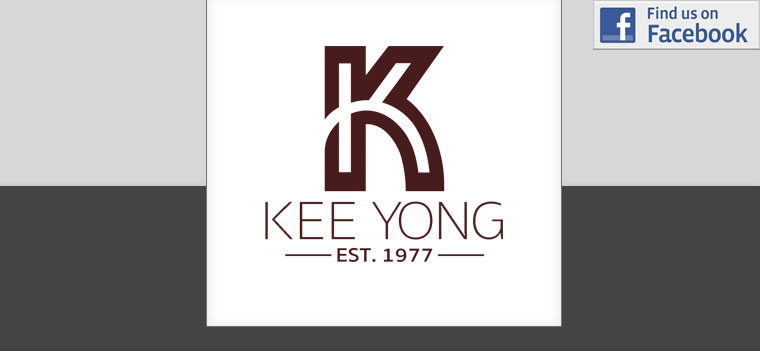The image features a horizontally bisected background, with the upper half in light gray and the bottom half in dark gray. Centered in this background is a prominent white square, nearly spanning the middle section. Dominating the white square is a very dark red, almost maroon, stylized 'K' logo with a thick border. Beneath the 'K', the name "KEE YONG" is displayed in capital letters. Further below, "EST. 1977" is flanked by lines on each side. In the top right corner of the image, a blue Facebook logo is accompanied by the text "Find us on Facebook," with "Find us on" in smaller font and both 'F's in 'Find' and 'Facebook' capitalized.